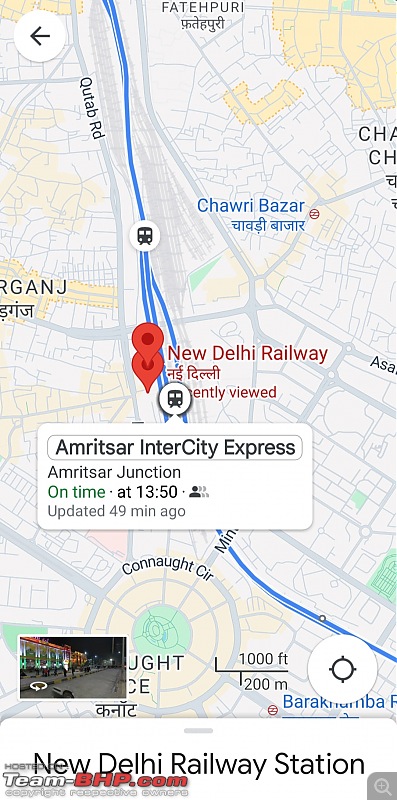The image depicts a detailed map with various elements and annotations. In the top left corner, there is a left arrow. The map contains multiple blue lines, likely representing bus routes. On the left, there is a label that reads "Kuta Broke," while the top of the map is marked with "Fateh Puri." Other notable locations include "Chari Bazaar" and "Khan Nakh Circle," a roundabout.

There are several colored annotations: red pen marks, and a section labeled "Amritsar Inner City Express," noting that the train is on time at 13:50 and that this information was updated 49 minutes ago. The map also includes a reference to "New Delhi Roadway."

At the bottom left, there are images showing the sky, grey ground, and a myriad of colorful lights. Scale indicators display measurements of 1,000 feet and 200 meters. A grey square is located at the bottom right, featuring a magnifying glass icon. Additionally, the map has a white line and some green markings, and there is a reference to "teen-php.com."